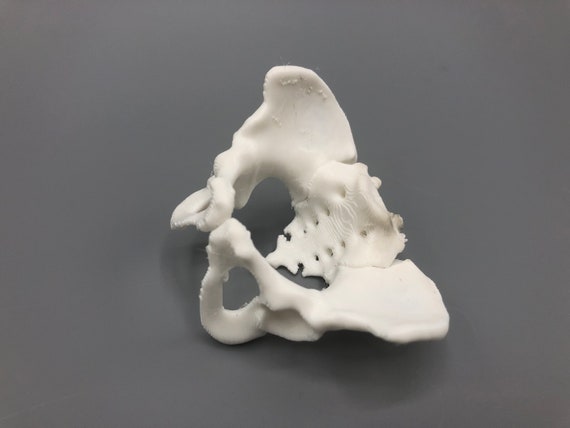The image showcases a detailed structure of a white pelvic bone, displayed against a gray background. The pelvis is oriented clockwise at roughly 45 degrees, with the top rim pointing towards the upper right corner of the picture. Both sides of the hip bone are prominently visible, along with the back sacrum which features four holes on each side for nerve passage. Additionally, there are two irregularly shaped areas resembling broken circles towards the edges. The tip of the tailbone and the frontal pubic bones, which have circular cutouts, are clearly visible. The gray background appears lighter in the upper left corner and darker in the lower right. The bone structure looks like a model or a cast rather than a real bone, likely utilized for scientific or educational purposes.